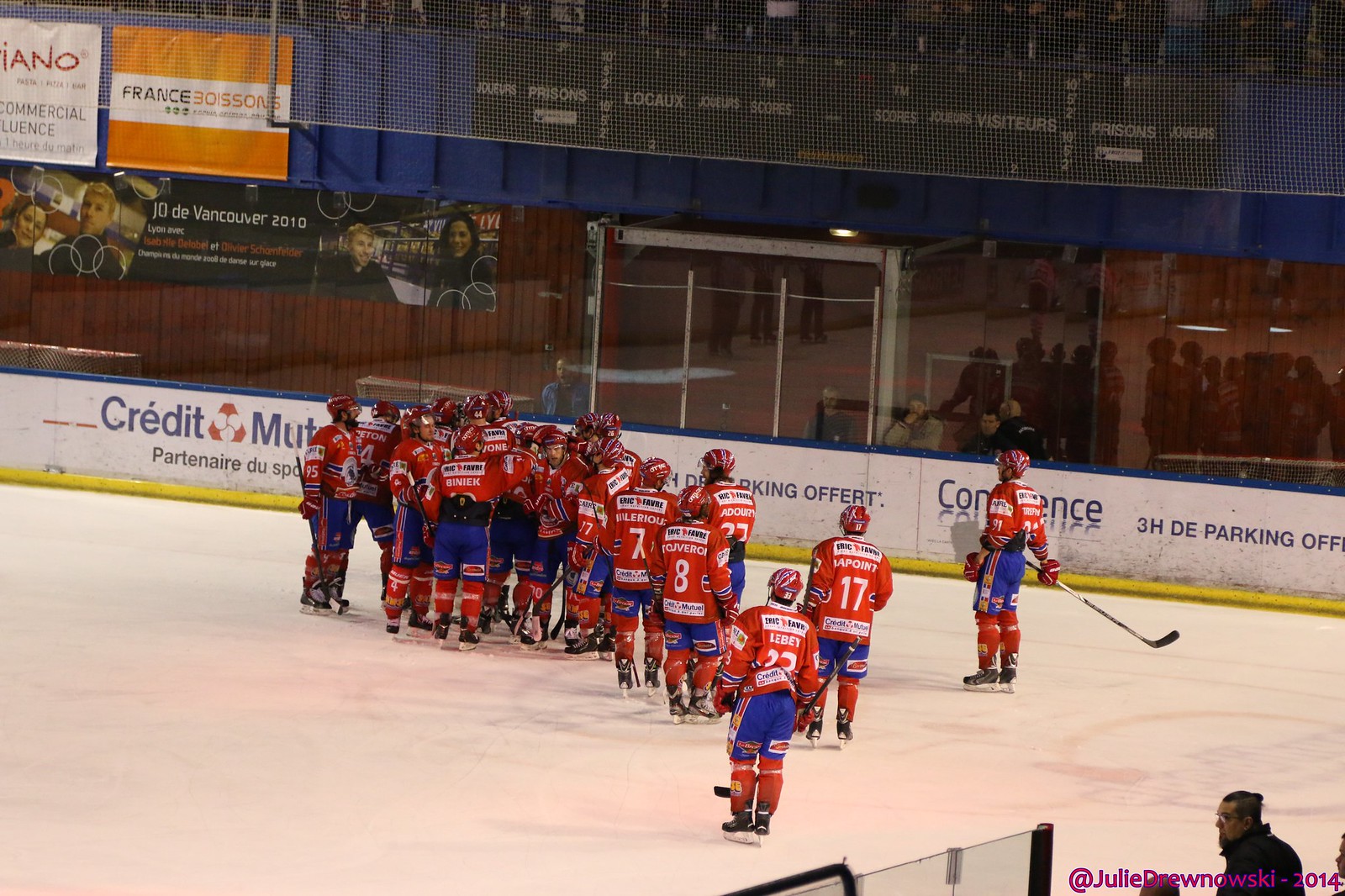The image depicts an indoor hockey arena with a group of ice hockey players gathered on the ice, indicating that it might be a practice session, a game that is about to begin, or that has just ended. The players are uniformly dressed in red tops with their names and playing numbers on the back, blue shorts, and red socks, complemented by red helmets. Surrounding the ice is a white-bordered outer wall adorned with various advertisements and sponsors in blue text, accompanied by a distinct yellow line at the bottom. Behind the glass barrier, there are a few spectators, particularly noticeable in the bottom right corner, as well as some heads seen scattered throughout the stands. Above, several banners and advertisements, including white, orange, and black banners, are visible alongside what appears to be a scoreboard. The year 2014 is mentioned in pink writing, further contextualizing the time frame of the event.